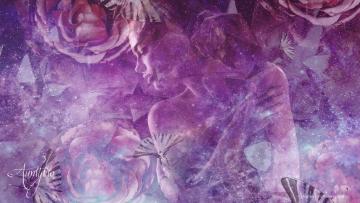The painting is a dreamlike, hazy composition primarily in shades of deeper purples, featuring a group of white and purple flowers, possibly roses, with faint abstract elements. Amidst this floral motif, a barely visible woman emerges from the background, as if viewed through a light fabric. She appears topless, with her arms crisscrossed over her chest, and is looking down towards the bottom left of the image, her eyes closed in a serene expression. The woman's form is delicately outlined, blending seamlessly with the flowers around her, which include larger petals to the left and smaller, partial flowers to the upper right. Additional whimsical details such as faint butterflies and floating seed pods reminiscent of dandelion seeds add to the ethereal quality of the artwork. In the bottom left corner, the artist's signature can be discerned.